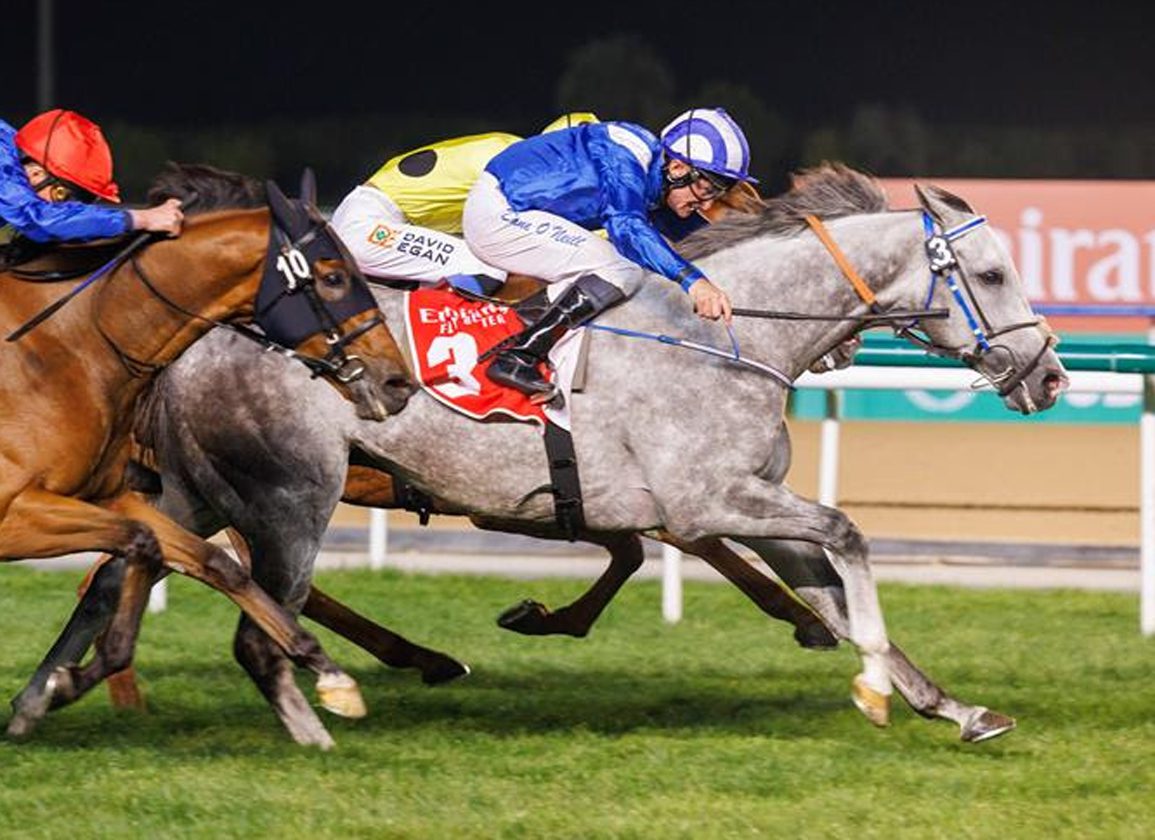In this nighttime scene at a horse race, three horses gallop from left to right across the frame. The foreground features a striking gray horse draped in a red banner labeled with the number three. Its jockey, dressed in blue silks and white pants, sports a blue and white striped helmet and black leather boots. Leaning forward over the horse's neck, he urges the horse onwards. To the left, partially visible, is a brown horse wearing a black face cover marked with the number ten. Its rider, also leaning forward intensely, wears a blue top and a red helmet. Behind these two, slightly obscured, is another brown horse with a rider donned in yellow silks featuring a black spot and white pants. Each horse's powerful stride captures the fierce motion of the race, their legs mid-air, hinting at the speed and intensity of the moment.